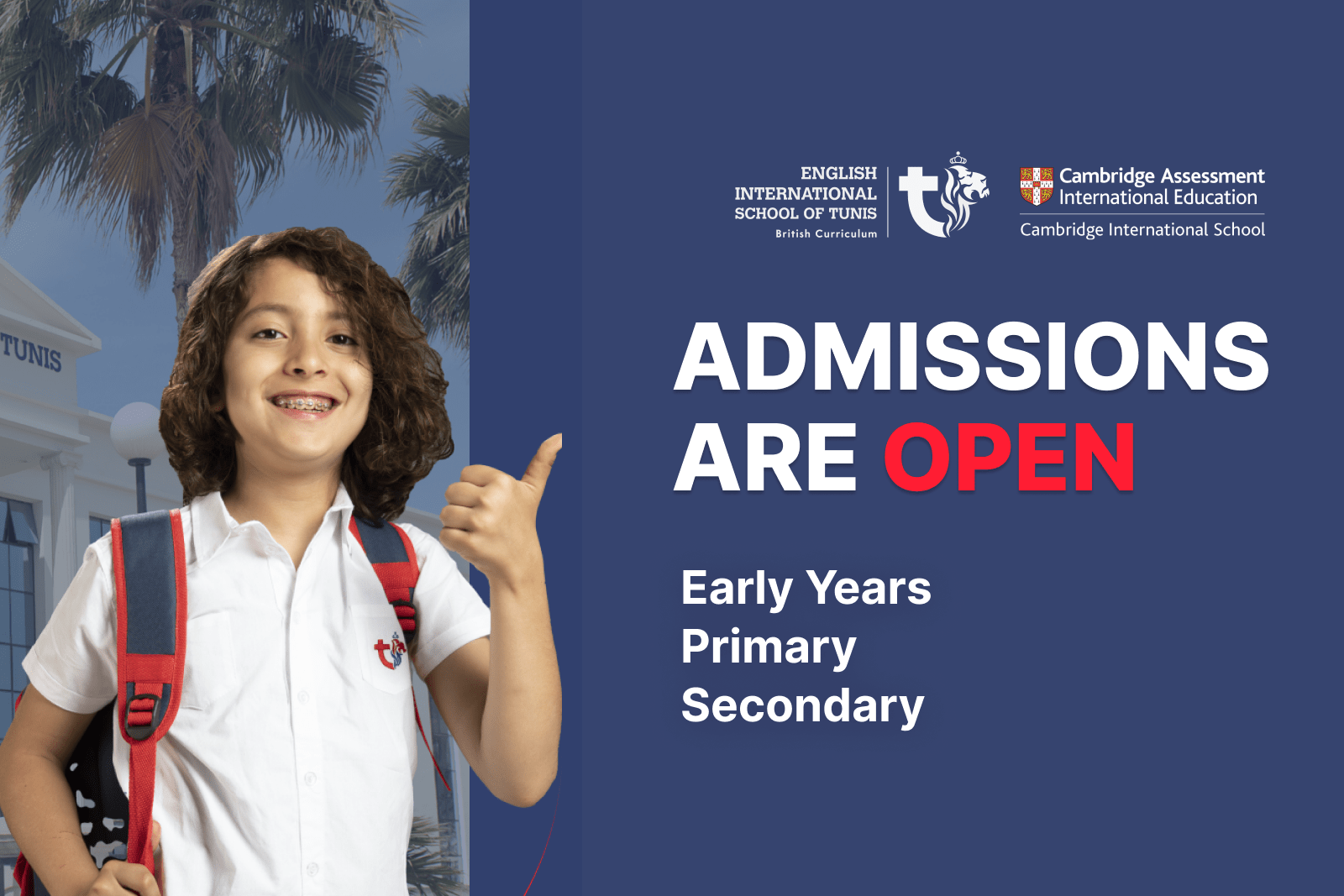A tall, rectangular image is divided into several distinct sections. The left third features a background with the tops of two tall palm trees reminiscent of those found in Florida. Only the top portion of these trees is visible, with the rightmost tree partially cut off.

Dominating the lower two-thirds of the image is a grinning Caucasian child, showcasing braces. The child, who appears to be a boy, sports a short, shoulder-length black hair and is dressed in a white, short-sleeved school uniform, adorned with a red and blue logo over the heart pocket. A red and blue backpack strap is visible, though the backpack itself is mostly out of sight. The child is giving a thumbs up gesture.

Behind the child is a white building with the inscription "Black Ladders Tunis" and tall white windows. Above the child's shoulder, a circular lamppost can be seen.

The right two-thirds of the image is dominated by a large blue box with various inscriptions in white letters. At the top, it reads "English International School of Tunis" in all caps, followed by "British Curriculum" in fainter white letters. Beneath this is a logo featuring a sideways "T" with the bottom curving to the right, crowned by a lion's head. To the right of the logo is a shield-like coat of arms with a white cross and four tan sections. Below this, the text reads "Cambridge Assessment International Education," followed by "Cambridge International School." A prominent white bar displays the word "Admissions," with the word "Open" in large red letters beneath it. The words "Early Years, Primary, Secondary" appear at the bottom in a smaller white font.